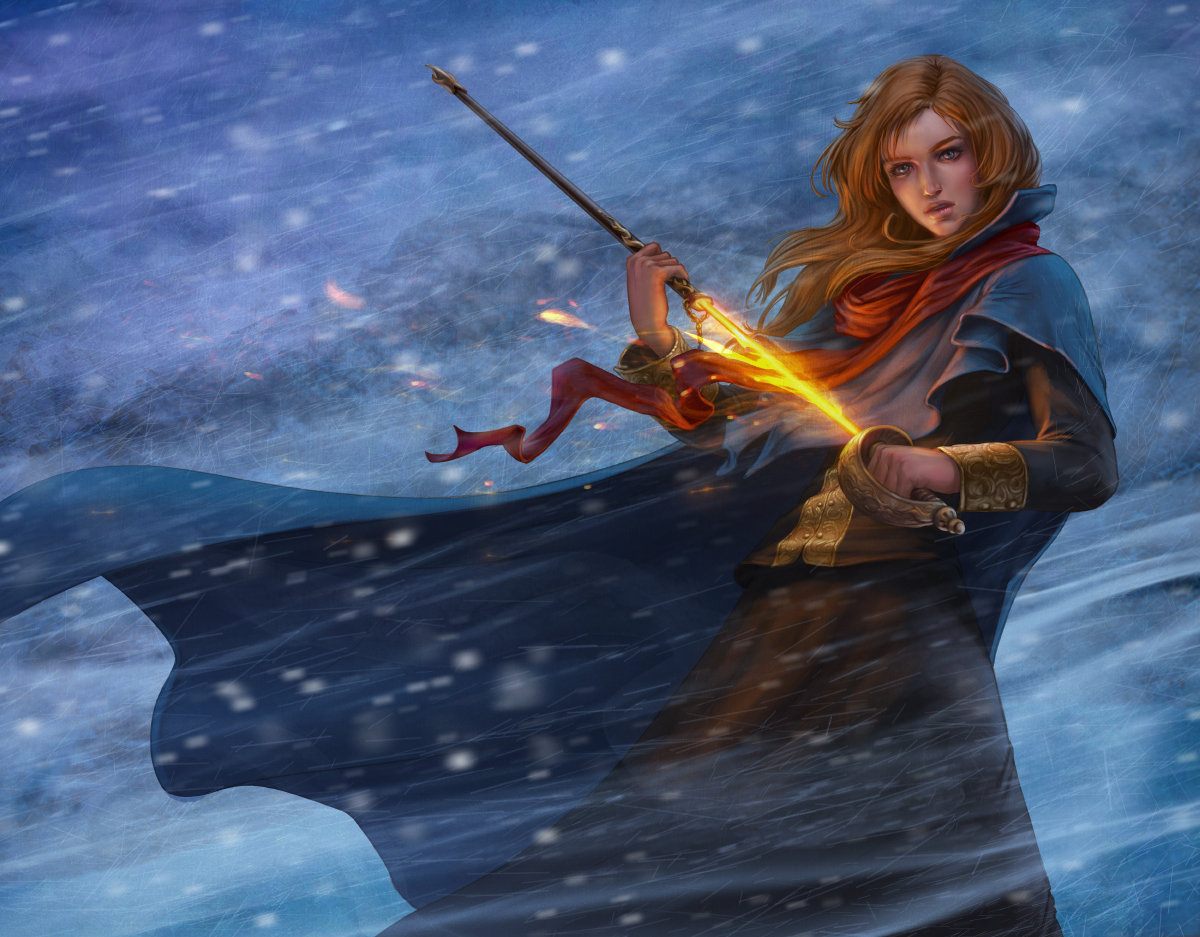In this striking sci-fi or fantasy image, a young female warrior with long, flowing reddish hair stands poised against a dynamic, swirly background. She wears a vibrant red cloak or scarf around her neck, which billows along with her long, flowing blue dress and a brown skirt beneath. Her right hand grasps the hilt of a sword, partially drawn from its sheath, with its tip ablaze with fire. The background swirls with hues of light and dark blue, interspersed with lines and specks of white and light blue, resembling stars or sparks in the air. The scene has a tempestuous, stormy atmosphere, with snow seemingly falling and a sense of the elements—wind and snow—swirling around her, evoking a sense of both magic and battle-readiness.